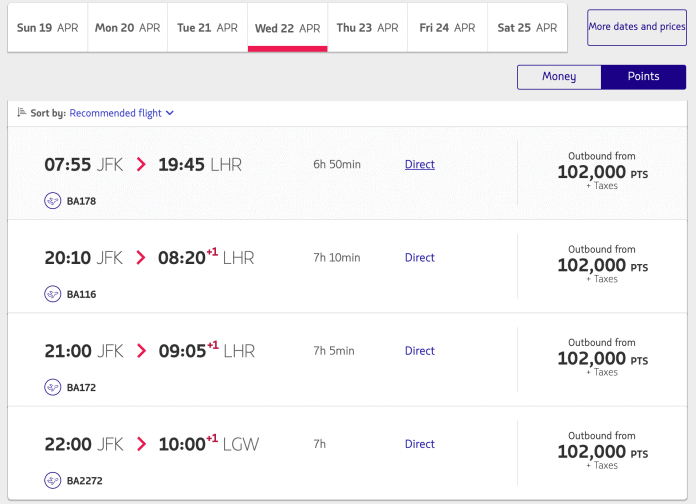This screenshot displays flight search results for airplane flights. At the top of the screenshot, a white bar showcases multiple date selections, ranging from Sunday, 19 April to Saturday, 25 April. The selected date, Wednesday, 22 April, is underlined in red. 

To the right of this white bar, there is a gray button labeled "More dates and prices." Below this bar, there are two buttons: one labeled "Money" and another labeled "Points." The flight results for Wednesday, 22 April, are displayed below these buttons, with the sorting option set to "Recommended."

The first of four flight options is detailed in a white rectangle. It shows a departure time of 07:55 from JFK (John F. Kennedy International Airport) and an arrival time of 19:45 at LHR (London Heathrow Airport). This flight is direct, with a duration of 6 hours and 50 minutes. The cost starts at 102,000 points plus taxes.

The second option listed below poses a departure time of 20:10 from JFK and an arrival time of 08:20 at LHR. This direct flight has a duration of 7 hours and 10 minutes, though specific pricing details are continued beyond the visible portion of the screenshot.